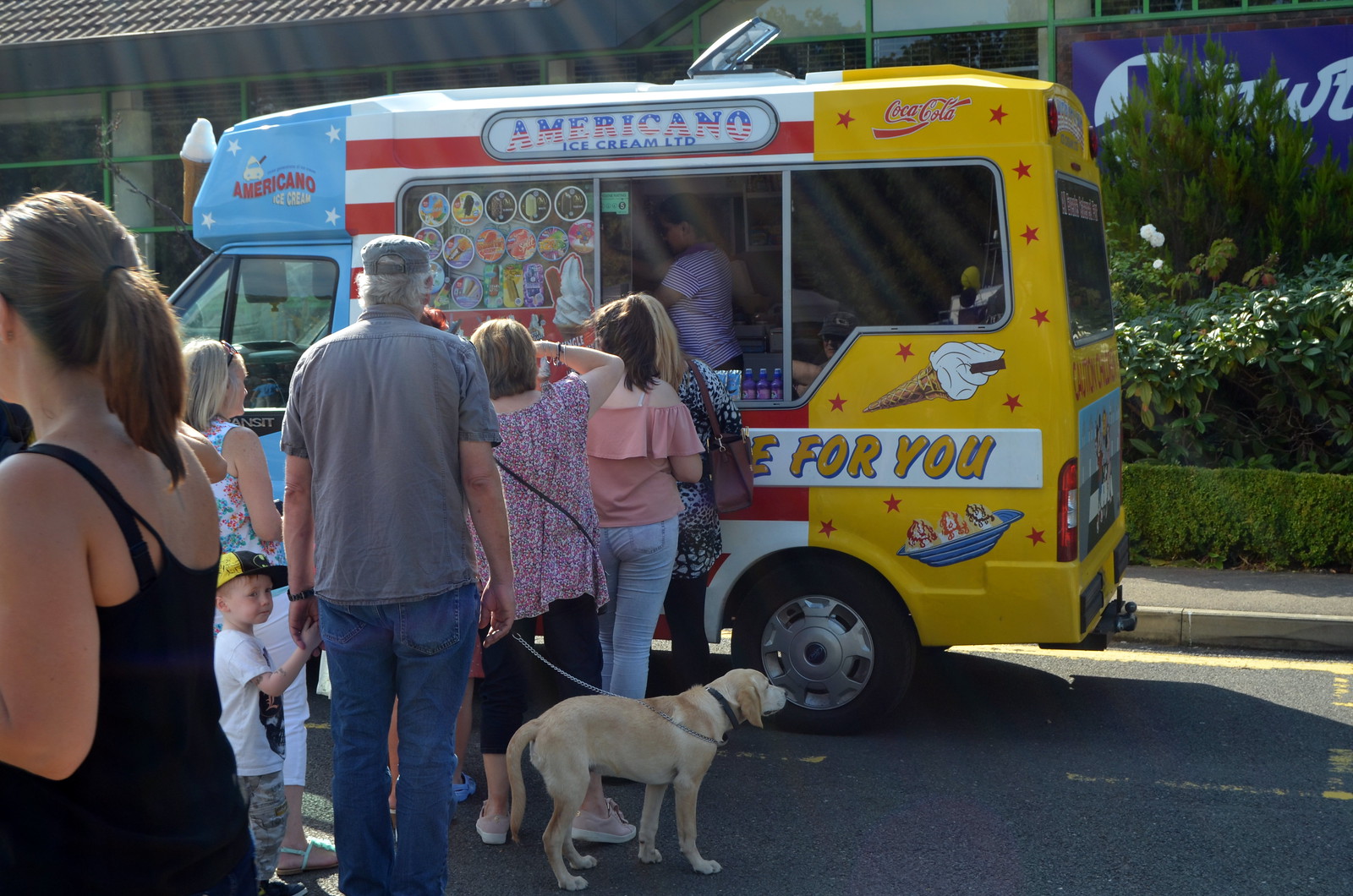The vibrant photograph captures a lively scene outside on a bustling street, featuring an eye-catching ice cream truck parked by the curb. The front of the truck is light blue, transitioning to white with red stripes in the middle, and finally yellow at the back. At the top of the truck's side, bold lettering reads "Americano Ice Cream Limited," accompanied by colorful icons like stars, an ice cream cone, and an ice cream sundae, along with a Coca-Cola logo on the right. The truck's sides boast large windows that are currently open, through which a woman can be seen preparing ice cream. 

A diverse group of around six people and a child forms an eager line in front of the truck, bathed in bright sunshine. At the forefront of the line is a woman in a black and white blouse, black pants, and holding a brown purse. Behind her stands a woman in a peach-colored blouse with blue pants, followed by another in a pink and purple blouse with a purse on her arm. Further down the line, a person holds a leash attached to a light brown dog, possibly a golden retriever, near the center-bottom of the image. The scene captures the anticipation and joy of a sunny day treat.